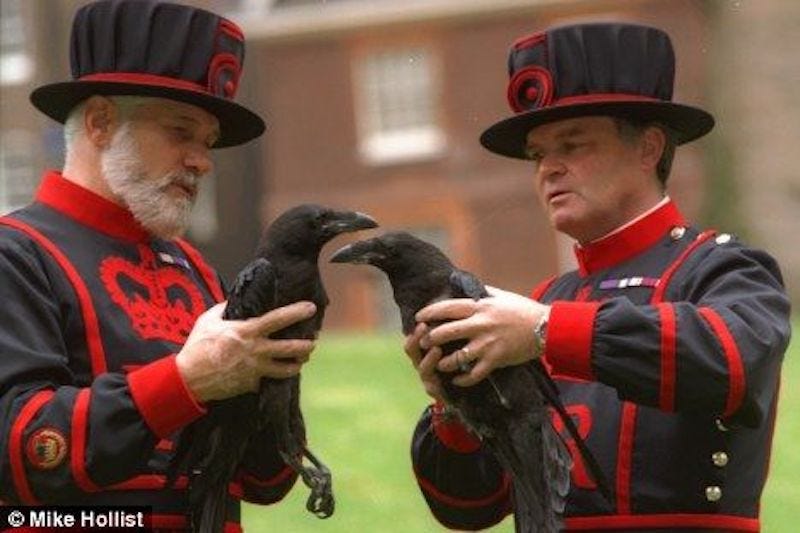In this daytime photograph set against the backdrop of a brick building and a field of grass, two senior men, presumably in their 50s or early 60s, stand facing each other. They are distinguished as British Yeoman Warders of the Tower of London, evident from their ceremonial black and red uniforms. Each uniform features a red-embroidered outline of a crown on the chest, white piping around the neckline, and red stripes on the sleeves. They complement their attire with black top hats adorned with red stripes near the base and a red circle in the center front. The man on the left, with white hair and a beard, and the man on the right, with short hair, both hold large ravens. The birds are positioned close to each other, almost touching beaks, as if they are examining or sniffing one another. Notably, a white text in the bottom left corner credits the photograph to Mike Hollist.